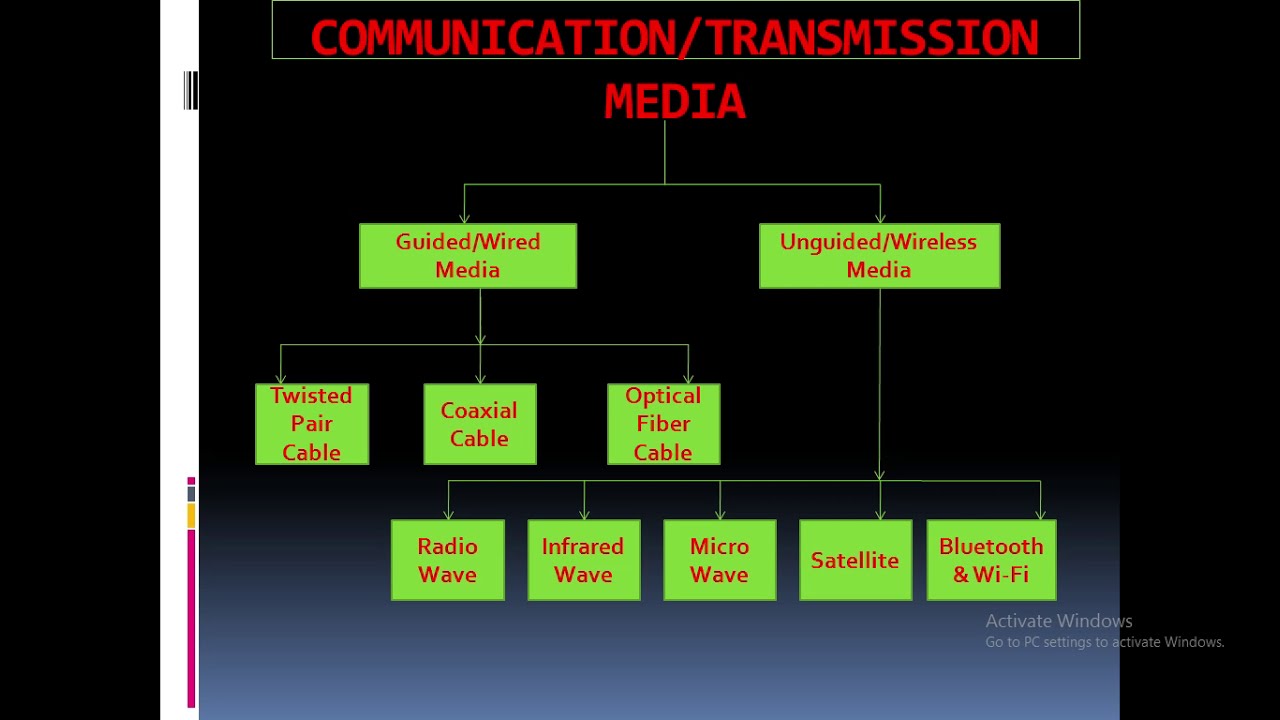The image is a detailed flowchart displayed on a predominantly black background, transitioning to a lighter blue towards the bottom. At the top, the title "Communication / Transmission Media" is written in red. A vertical white bar runs down the left side, giving structure to the design. The flowchart itself is composed of lime green blocks with red text. It branches into two main categories: "Guided / Wired Media" on the left and "Unguided / Wireless Media" on the right.

Under "Guided / Wired Media," there are three subcategories—each in a green block—labeled "Twisted Pair Cable," "Coaxial Cable," and "Optical Fiber Cable." On the "Unguided / Wireless Media" side, there are five subcategories: "Radio Wave," "Infrared Wave," "Microwave," "Satellite," and a combined category of "Bluetooth and Wi-Fi."

Additionally, in the lower right-hand corner, a white text reminder reads, "Activate Windows. Go to PC settings to activate Windows." This suggests the image was captured on a computer screen that requires activation, possibly indicating its use as a reference or instructional material for networking technologies or internet connectivity concepts.